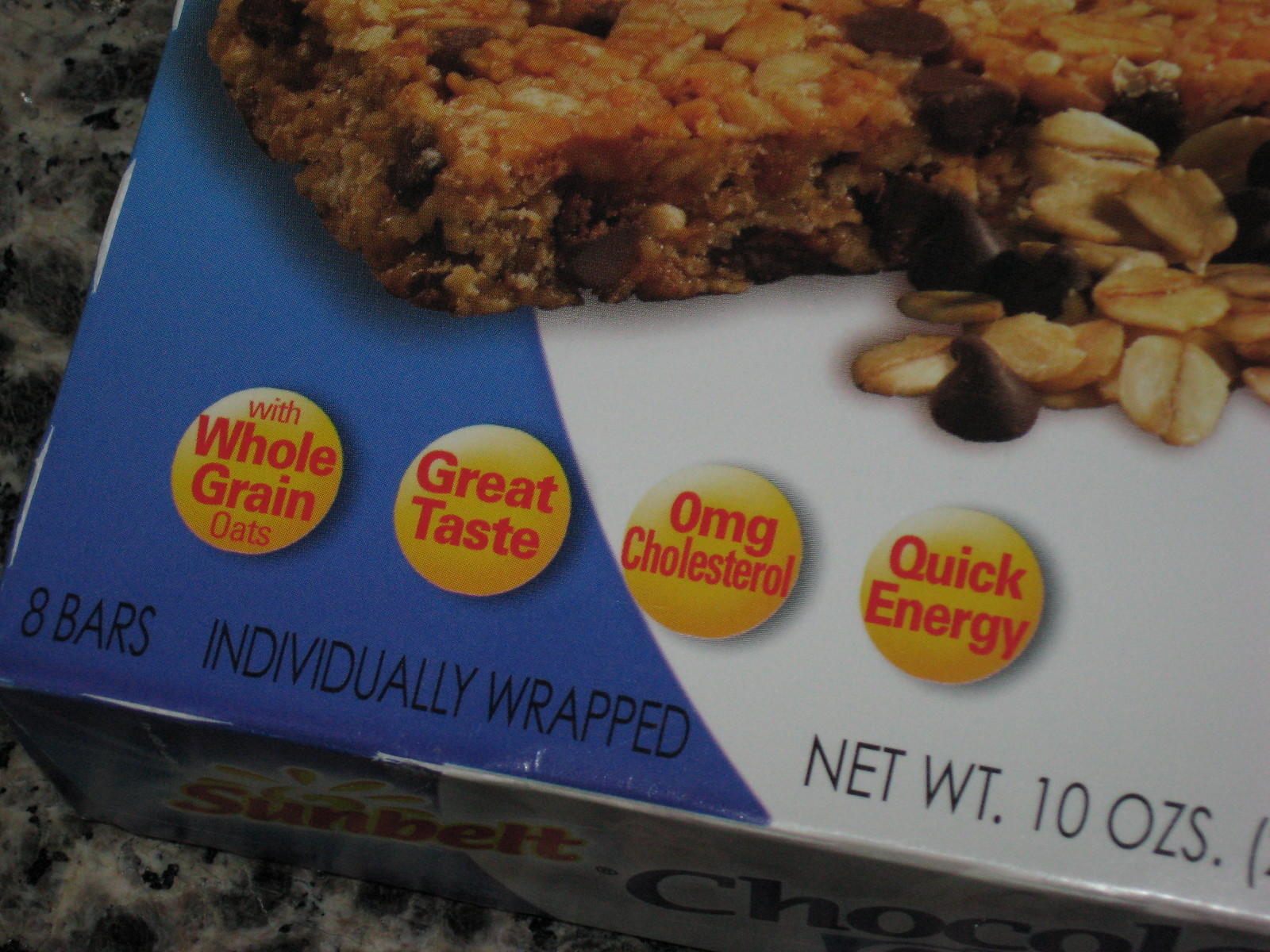This close-up photograph depicts the bottom left corner of a granola bar box. The packaging has a gradient transitioning from dark blue to white. The bottom text reads, "Eight bars individually wrapped," followed by "Net WT. 10 OZ," and further details partially cut off by the image edge. Prominent on the box are four circular yellow icons with red text, stating: "With Whole Grain Oats," "Great Taste," "Zero Milligrams of Cholesterol," and "Quick Energy." A highly detailed and enlarged image of a textured granola bar adorned with chocolate chips and oats is prominently displayed. Additionally, the Sunbelt logo, featuring a red background with a small yellow sun, is visible. The bar itself is a mix of light brown and golden grains interspersed with dark chocolate chunks, shown alongside chocolate pieces and oats presented in higher detail. The box rests on a light gray countertop speckled with black and dark gray spots.